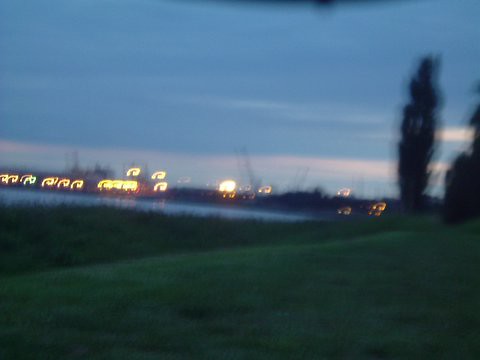This outdoor photograph, captured around twilight or early morning, showcases green rolling hills with two prominent hills in the foreground. To the right, a couple of tall, narrow trees rise up, alongside a blurry roadway that exhibits motion blur from oncoming traffic headlights. These headlights possibly include larger vehicles like transfer trucks, identifiable by higher-positioned lights. To the left on the horizon, you can see the scattered lights from buildings. The sky is cloudy, bathed in blue shading with streaks of light suggesting either a rising or setting sun. The entire scene appears slightly out of focus, contributing to a dreamy, tranquil atmosphere. In the immediate foreground, there is green grass, possibly mingling with some grassy weeds near a barely visible edge of water, adding to the natural beauty of the landscape.